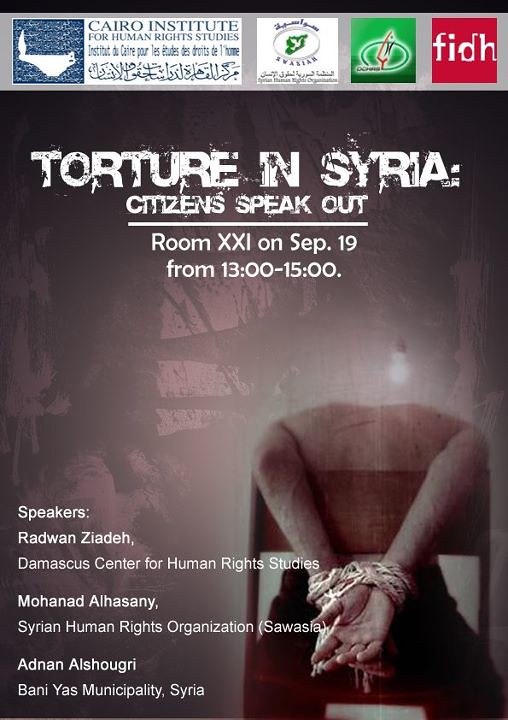This is an advertisement for an event titled "Torture in Syria: Citizens Speak Out," scheduled to take place in Room XXI on September 19th from 1300 to 1500 hours. The top of the flyer features promotional logos, including the Cairo Institute for Human Rights Studies. The bottom right corner of the advertisement shows a poignant image of a person tied to a chair, their head obscured, with their hands bound behind their back. On the bottom left, in white font, the advertisement lists the speakers: Radwan Ziadeh from the Damascus Center for Human Rights Studies, Mohanad Al Ahansi from the Syrian Human Rights Organization, and Adnan Al-Shugri from Bani Yas Municipality. These individuals are presumably set to testify about the torture occurring in Syria.